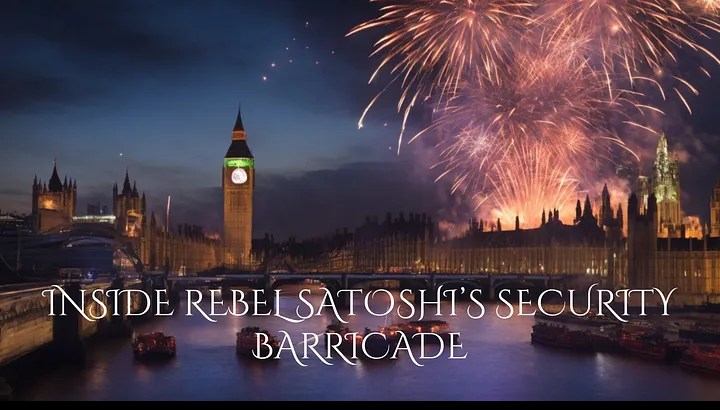This is a vibrant, color photograph taken at night, showcasing an iconic London scene. Dominating the backdrop is Big Ben, majestically illuminated and surrounded by other famous London landmarks near the Thames River. A dazzling array of pink and yellow fireworks light up the sky, suggesting a celebratory event, possibly for New Year's or another significant occasion. The text "Inside Rebel Satoshi Security Barricade" is prominently displayed across the bottom in flourishy white print, indicating it could be part of an advertisement or thematic event, potentially linked to cryptocurrency. The sky, while mostly clear, features a few visible stars, including what seems to be the Big Dipper. In the harbor, several boats are anchored, their occupants pausing to admire the spectacular fireworks display. The overall scene captures the festive spirit and grandiosity of the moment, making it resemble an idealized postcard of London at night.